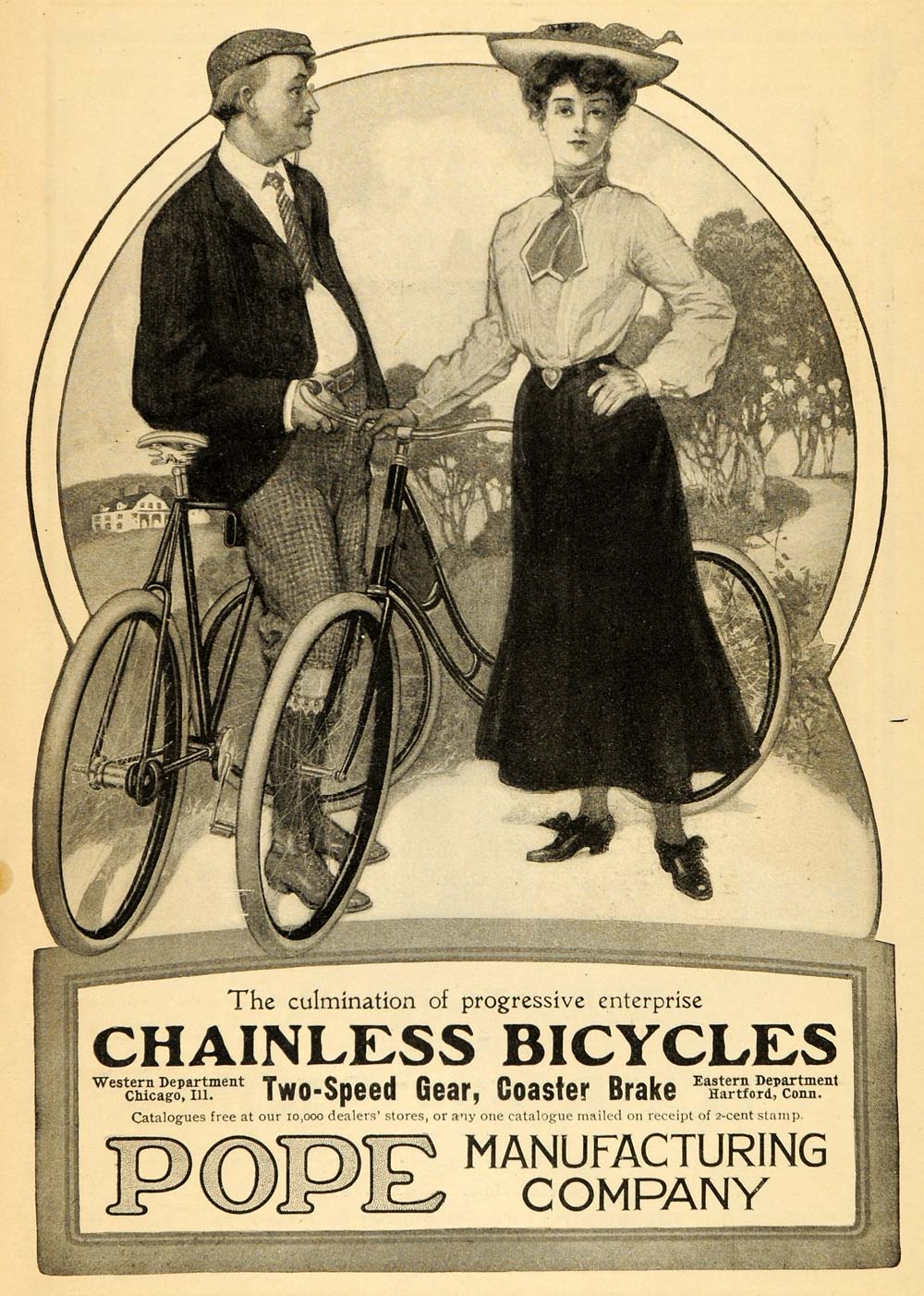The image depicts a vintage black-and-white advertisement banner. At the center, a man and a woman stand next to their bicycles, evoking an early 1900s era. The man, with brown hair and a mustache, wears a black suit jacket over a striped tie, knee-length pants, boots, and a cap. The woman, with brown curly hair, sports a white blouse, black skirt, black shoes, and a scarf around her neck. She also balances a tray with a bird on her large hat. Both figures are depicted in a postured stance against a backdrop of trees. Prominently displayed text below them reads, "The culmination of progressive enterprise, chainless bicycles, two-speed gear, coaster brake." Beneath this, the advertisement notes "Pope Manufacturing Company" and mentions catalog availability free at 10,000 dealer stores, or via mail for two cents.